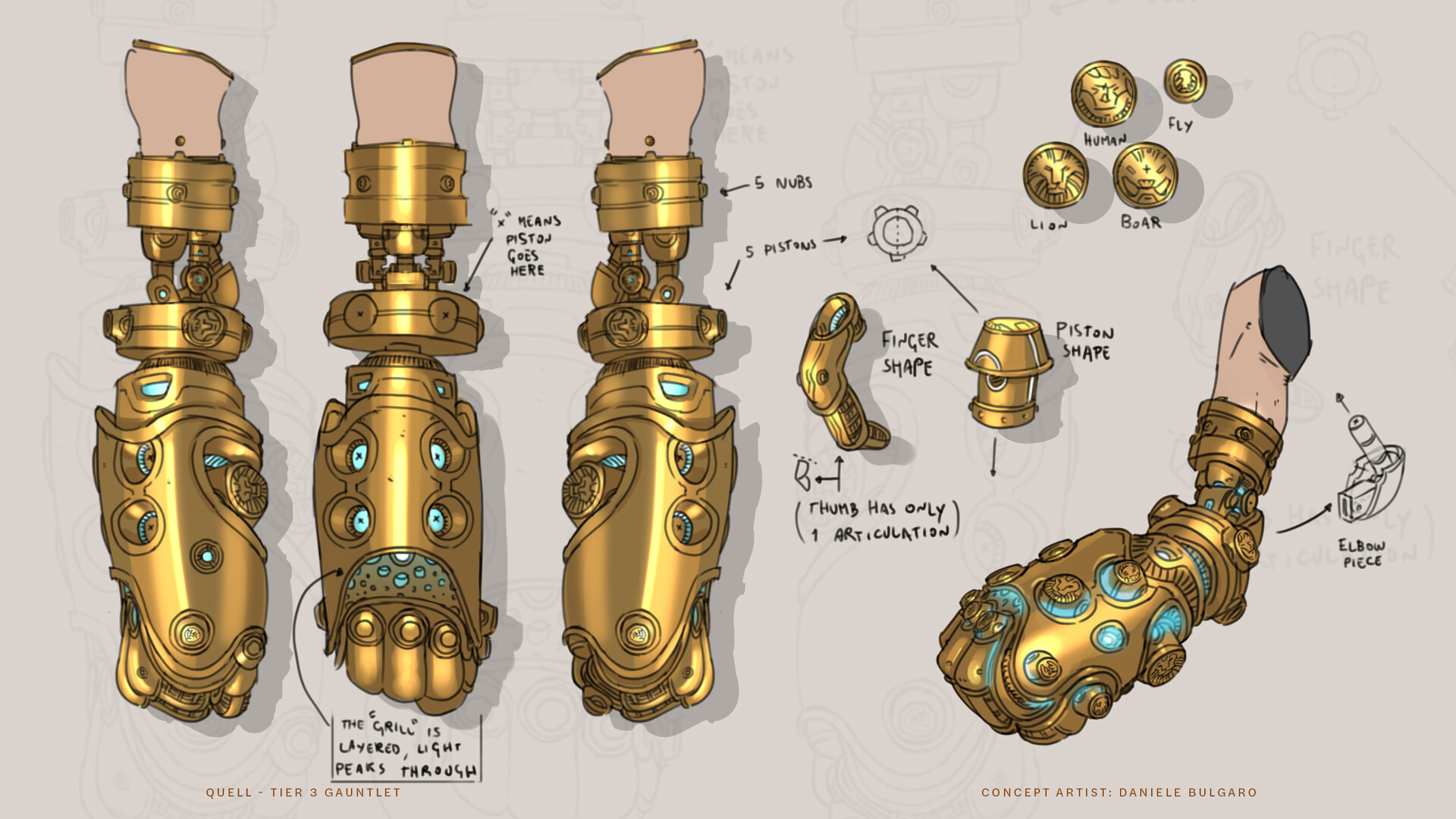The image depicts a highly detailed conceptual drawing of a mechanical prosthetic arm, labeled as the "Quell Tier 3 Gauntlet." Designed by concept artist Danielle Bulgaro, the prosthetic features a gold or brass coloration with teal accents and some hints of brown. The central piece showcases an arm equipped with an elbow segment, surrounded by three separate components on the left. Arrows indicate various parts of the appendages, such as piston and finger shapes, highlighting the mechanical intricacy.

The left section of the image presents the prosthetic from three perspectives: front, side, and back, offering comprehensive views of its design. To the right, a detailed illustration shows the attachment points to the elbow and forearm, and an array of buttons adorned with different symbols, including human, fly, lion, and boar. The artwork is noted for its professional quality, showcasing the golden metallic finish complemented by blue teal lights and detailing.